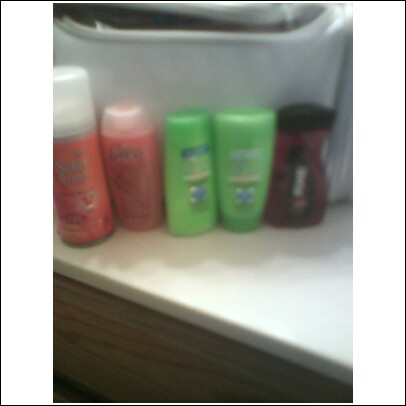In this blurry photograph taken inside a bathroom, we see five toiletry items arranged in a row on a white countertop. Below the countertop is a partially visible dark brown wooden cabinet. Starting from the left, the first item appears to be a bottle of shaving cream, characterized by its pink label and translucent white cap. Next to it is a similarly colored pink bottle, likely containing lotion, with an oval shape and a clear top. In the center of the lineup are two green bottles, one tapered towards the top and the other towards the bottom, suggesting they are shampoo and conditioner. The green color is described as foamy or lime. The item on the far right is a dark purple bottle with a black cap. Behind these toiletries, a grayish bag made of soft material is partially visible. The image is cropped closely, adding to the difficulty in precisely identifying the items.